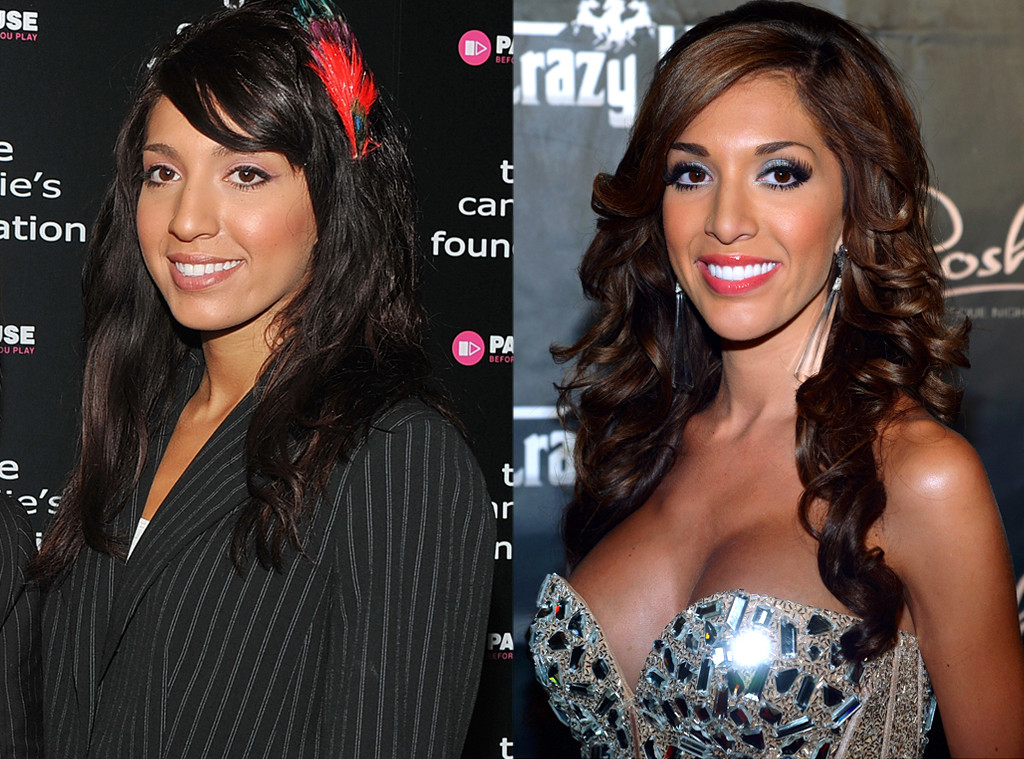The image features two side-by-side photographs showcasing the transformation of Farrah Abraham from "Teen Mom." The left photograph, taken during her younger years, depicts her with long, dark hair adorned with a red feather. She is seen smiling and wearing a black pinstripe suit jacket over a white top, with highlights like a red feather in her hair, standing against a black backdrop with white text that is somewhat obscured but includes partial words such as "FOUNDATION" and "CAN." 

Contrastingly, the right photograph portrays an older Farrah, her appearance significantly altered, possibly due to cosmetic enhancements. She sports a much fuller hairstyle with added highlights and wears heavy eye and lip makeup. Her attire is a striking, low-cut, gold dress embellished with chunky rhinestones or crystal pieces, complementing her large, silver earrings. This image also features a black background with white text, although much of it is obscured by her presence. The color palette across the image includes shades of black, white, gray, silver, blue, pink, red, and various browns, capturing the stark differences in her appearance over time.